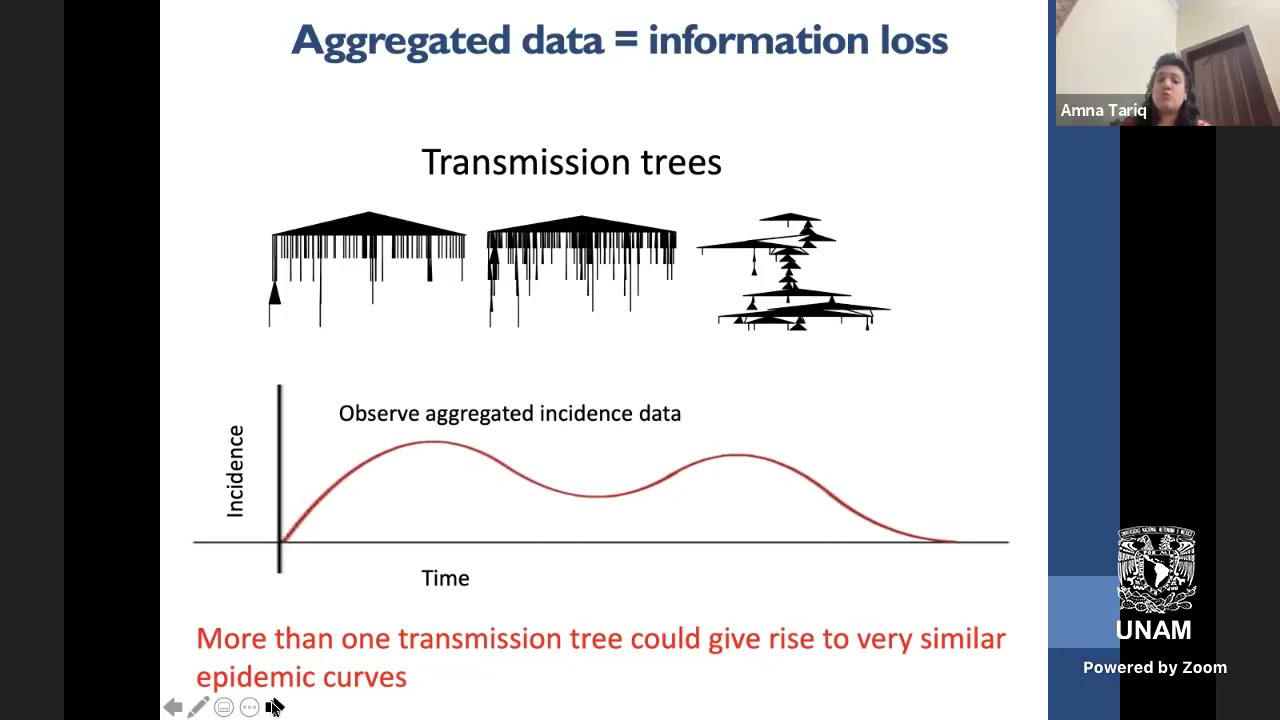The image is a screenshot from a Zoom presentation, primarily showing a slide titled "Aggregated Data Equals Information Loss." The slide occupies most of the frame, flanked on the far left and right by dark gray and black stripes, along with an additional blue stripe on the right. Positioned in the top right corner of the slide, there's a photograph of the presenter, Amna Tariq, with her name labeled underneath. She has long, shoulder-length black hair and is seated in a room with white walls and a door behind her.

The main slide consists of the title in blue text, followed by the subtitle "Transmission Trees" in black print. Below this are three distinct diagrams; the first two resemble triangles with various straight lines extending downward, representing different lengths. The third image appears as irregular zigzag lines. Below these diagrams is a graph labeled "Observe Aggregated Incidence Data," with "Incidences" written vertically and "Time" written horizontally. The graph itself features a red line with two prominent humps. At the bottom of the slide, in red print, it states, "More than one transmission tree could give rise to very similar epidemic curves."

The lower-right corner of the image includes a logo with the letters "UNAM" beneath it, accompanied by the phrase "powered by Zoom." The UNAM logo appears to feature two eagles back-to-back, with the continent of South America contained within a shield between them. This detailed and multi-layered presentation slide emphasizes the complexities of data aggregation and its potential impact on information clarity.